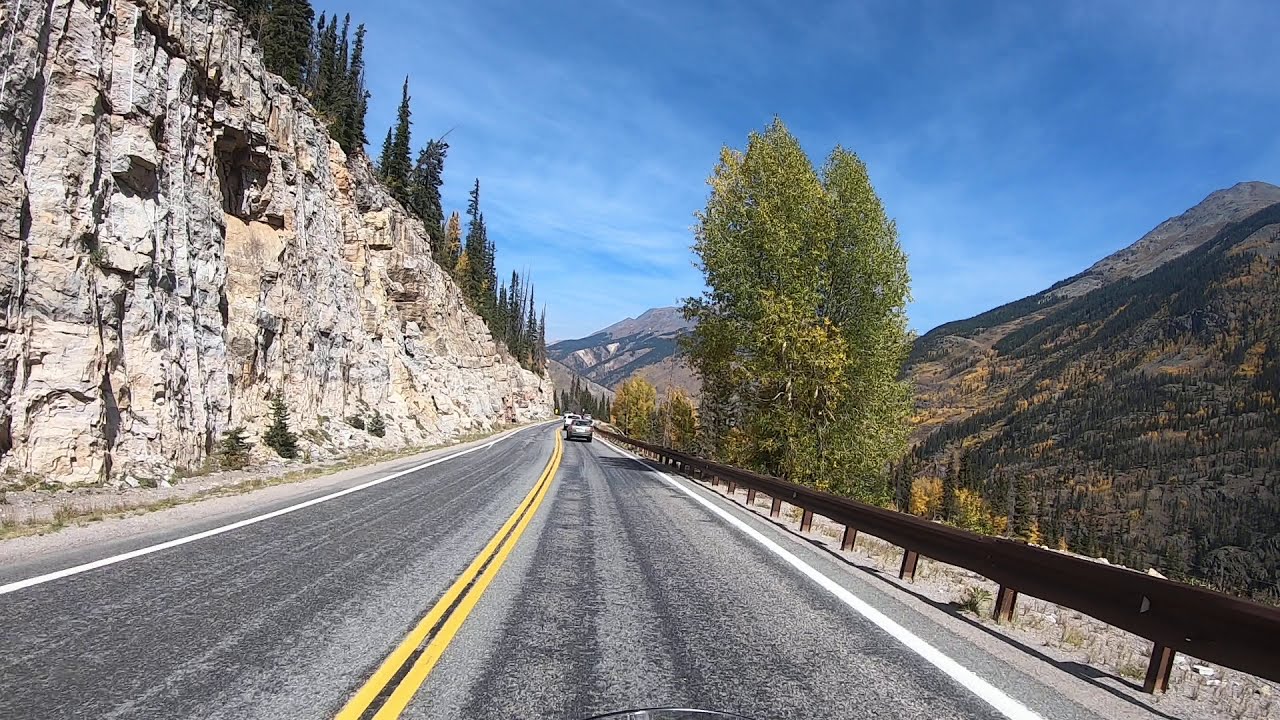The photograph is a wide rectangular image depicting a two-lane highway snaking through a mountainous region. The road, paved in gray with a solid double yellow line in the center and bordered by solid white lines on either side, starts prominently at the bottom and recedes into the horizon at the middle of the image. On the right side, the highway is flanked by a short brown metal guardrail, beyond which a lush green hill descends before rising into a vast mountain range dotted with tall, dark green pine trees. The left side is dominated by a steep, jagged rock face in shades of light gray and tan, capped with a row of narrow, towering pine trees. The sky above is a clear, light blue with thin, wispy white clouds, indicating a bright, sunny day. Vehicles, perhaps two or three, can be seen faintly in the distance on the right lane, driving away from the camera toward the horizon, suggesting the photograph might be taken from the back of another moving car. The composition and sharp contrast of natural elements lend the scene a majestic quality.